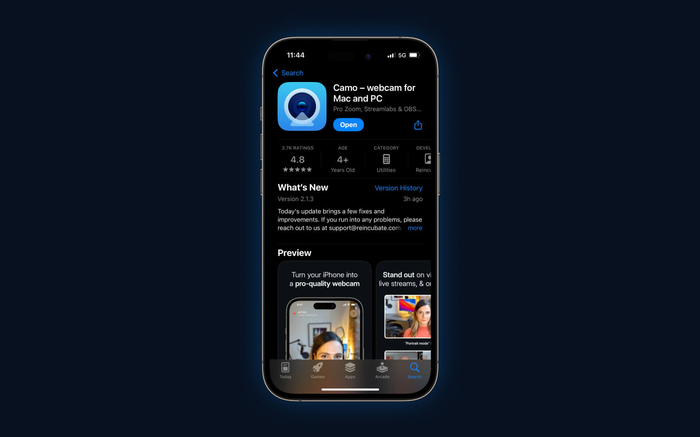In the background of the image, it is quite dark. On the top left corner of a smartphone screen, the time reads 11:44, and there are indicators showing three out of four signal bars, 5G connectivity, and a full battery. A blue square with a camera icon signifies a search function. To the right, there is text that reads "Camo - Webcam for Mac, PC, P.O. Zoom, Streamlabs, and OBS. Open." highlighted in blue. 

The screen shows a rating of 2.7K with 4.8 stars, indicating its popularity. The app is suitable for ages 4 and above and falls under the utility category with the developer noted. The latest update is version 2.1.3, released three hours ago, bringing a few fixes and improvements. Users are prompted to contact support at reincubate.com if they encounter any issues. The text also mentions "Retext as previewed. Turn your phone into a pro quality webcam," suitable for video and live streams.

At the bottom left of the screen, there is an icon for "Phone" labeled "Today". Next to it is a "Games" icon depicting a rocket ship, and an "Apps" icon showing squares stacked on each other. Additionally, there is an "Arcade" icon with a stick figure emerging from an object. A blue magnifying glass icon for search can also be seen. 

The bottom bar has a blurry background with the majority of the image appearing black, with white or silver edges.